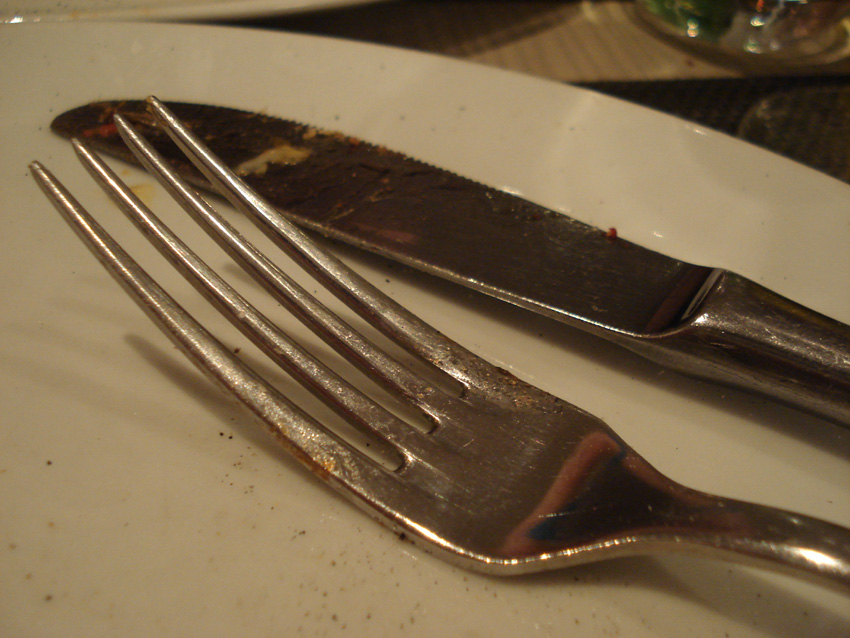The image is a detailed close-up of dirty silverware resting on a white ceramic plate, captured from the top left corner, arcing down to about an inch beneath the opposite side. Prominently, a long-tined dinner fork stretches diagonally from the right, its tips reaching towards the upper left. Alongside it, a stainless steel dinner knife, with a dull edge facing the plate, lies parallel. Both utensils are coated with remnants of food, possibly yellow and crusty like eggs, and appear greasy with some crumbs or black specks scattered around. The white plate looks either textured or simply dirty with a greasy appearance. In the barely visible background at the top right, there's a hint of a wooden table and possibly a napkin or placemat. Additionally, an indistinct outline of a drinking glass and perhaps a menu or another object subtly fades into the background, adding an evocative, abandoned atmosphere to the scene.